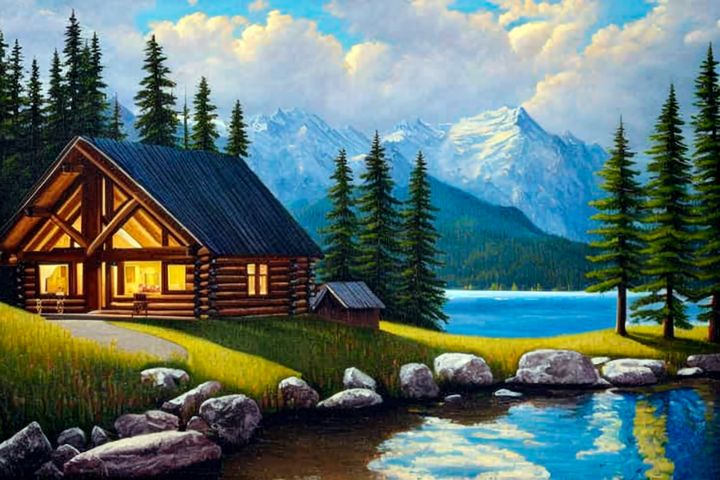This illustration depicts a tranquil mountain scene with a cozy log cabin positioned to the left of the image. The cabin, characterized by its dark roof and luminous yellow glow from its many glass windows, sits in a small grassy clearing. A narrow, gray stone path leads from the cabin's entrance to a nearby pond surrounded by large, smooth gray rocks. This pond, reflecting the blue sky and puffy white clouds, extends towards the right of the foreground.

Adjacent to this pond and separated by a strip of land, lies a larger, turquoise-blue lake. The reflective surface of this second body of water mirrors the surrounding environment, which includes towering pine trees and a landscape of green, rolling hills.

In the background, majestic snow-capped mountains rise, their rocky, turquoise-tinged faces partially forested at the lower levels. The sky overhead is a vibrant cerulean blue, dotted with clusters of billowing white clouds. The scene exudes peacefulness and serenity, with the detailed interplay of natural elements and the rustic warmth of the cabin inviting viewers to imagine the quiet solitude of this idyllic mountain retreat.